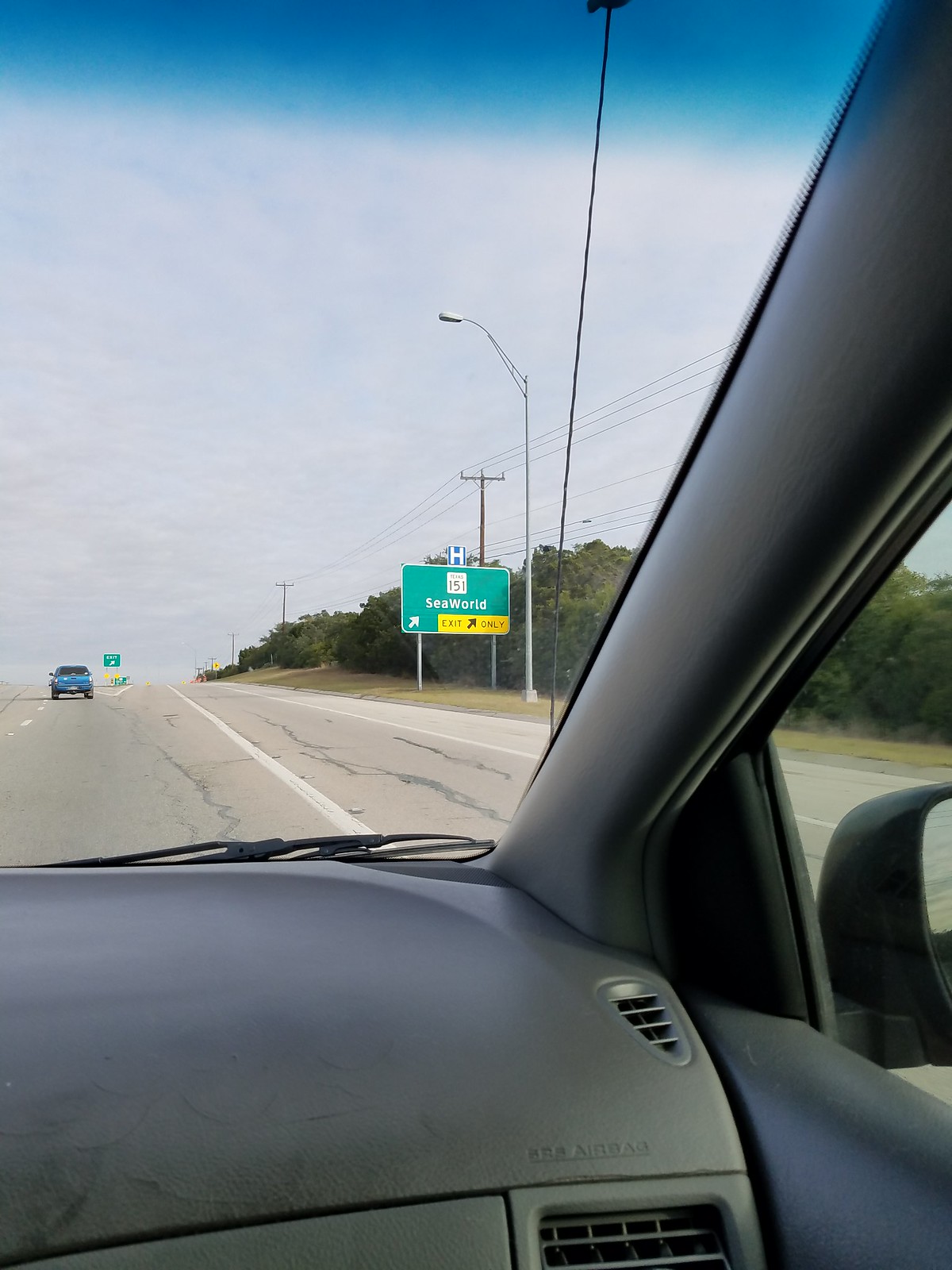This detailed image captures the view from the interior passenger seat of a car with a gray interior, looking out through the front and part of the side window. The scene unfolds on a highway under a daytime sky that is mostly blue with a haze of white clouds. Ahead, there is a large green freeway sign adorned with white lettering that indicates an exit to SeaWorld. The sign features a mix of directional symbols: diagonal right arrows, a route number 151, a blue "H" for hospital, and an "Exit Only" caution noted in yellow and black with an upward 45-degree angle arrow. To the right of the road, tall street lights and power lines run parallel to a paved shoulder area, flanked by lines of green trees. Notably, a blue car is visible ahead in the right lane, approaching the exit for SeaWorld, further contributing to the sense of an active journey along this off-gray paved road, marked with white lines. The dashboard's edge and a small portion of the passenger side mirror are also visible, grounding the viewer inside the vehicle.